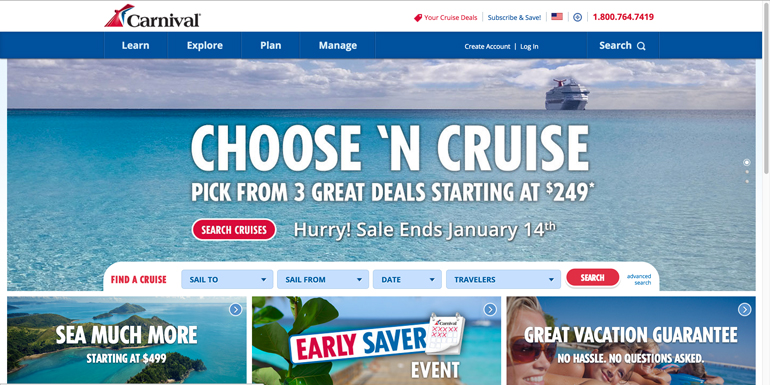**Carnival Cruise Lines Webpage Screenshot**

At the top left corner of the image, the Carnival Cruise Lines logo and the word "Carnival" are prominently displayed. Across the top of the screenshot, there is a white navigation bar featuring options for "Your Cruise Deals," "Subscribe and Save," an American flag icon, a plus sign inside a blue circle, and a phone number in bold red text: 1-800-764-7411.

Directly below the white navigation bar is a blue bar with white text menu options for "Learn," "Explore," "Plan," "Manage," "Create Account," and "Log In." To the right is a search bar option.

The main section of the image showcases a panoramic photograph of a serene, still blue ocean under a sky adorned with white clouds. A massive cruise ship is visible in the distant horizon heading towards the viewer. Overlaid on this image, in white text, is the phrase "Choose and Cruise, pick from three great deals starting at $249," alongside a red "Search Cruises" button. Additional text, "Hurry, Sale Ends January 14th," appears in white letters.

Below this main image, search options are provided, including "Find a Cruise," "Sail To" (with a dropdown menu), "Sail From" (dropdown menu), "Date" (dropdown menu), "Travelers" (dropdown menu), a red "Search" button, and a blue text link for "Advanced Search."

Further down, three smaller photographs are presented:
1. The first image shows lush green islands surrounded by the sea with the text "See Much More" (spelled as "S-E-A Much More") and a starting price of $499.
2. The middle image features a beach scene with sand and a green plant with broad leaves in the foreground. Overlaid text highlights an "Early Saver Event" with a calendar graphic showing some dates marked with an X.
3. The rightmost photograph depicts four tanned individuals, some wearing sunglasses, lounging on a beach with the ocean and greenery visible in the background. Superimposed text reads "Great Vacation Guarantee, No Hassle, No Questions Asked."